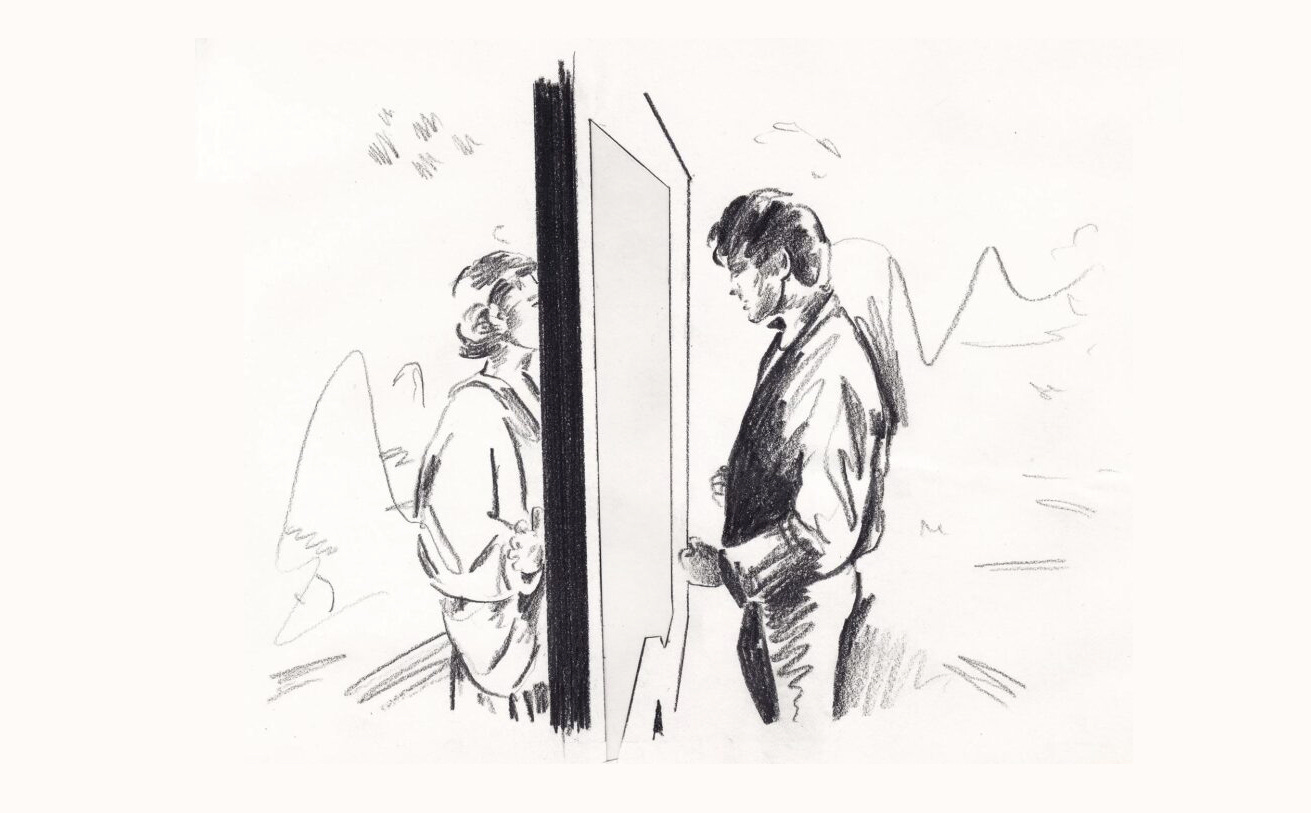This detailed black-and-white pencil sketch, set against an off-white background, vividly recalls the iconic scene from A-ha's "Take On Me" music video. Central to the composition is a plain white door seen in side profile, with visible door frame lines defining its shape. The door stands between a sketched man and woman, each positioned on either side and seemingly poised to meet. The woman, drawn with light hair that falls to her neck, has an ethereal presence reminiscent of an angel, possibly due to her robe-like attire and the overall sketch aesthetic. On the right side, the man resembles Elvis Presley with his distinctive slicked-back black hair, some strands falling over his forehead. His outfit features tight-fitting pants and a slightly loose jacket around the shoulders, embellished with curvy, illustrative lines. Both figures are outdoors, as suggested by the abstract, curvy pencil strokes filling the background, adding a dynamic, almost whimsical atmosphere to the scene. Their gazes are fixed on each other, emphasizing the emotional tension and anticipation of their impending encounter through the door.